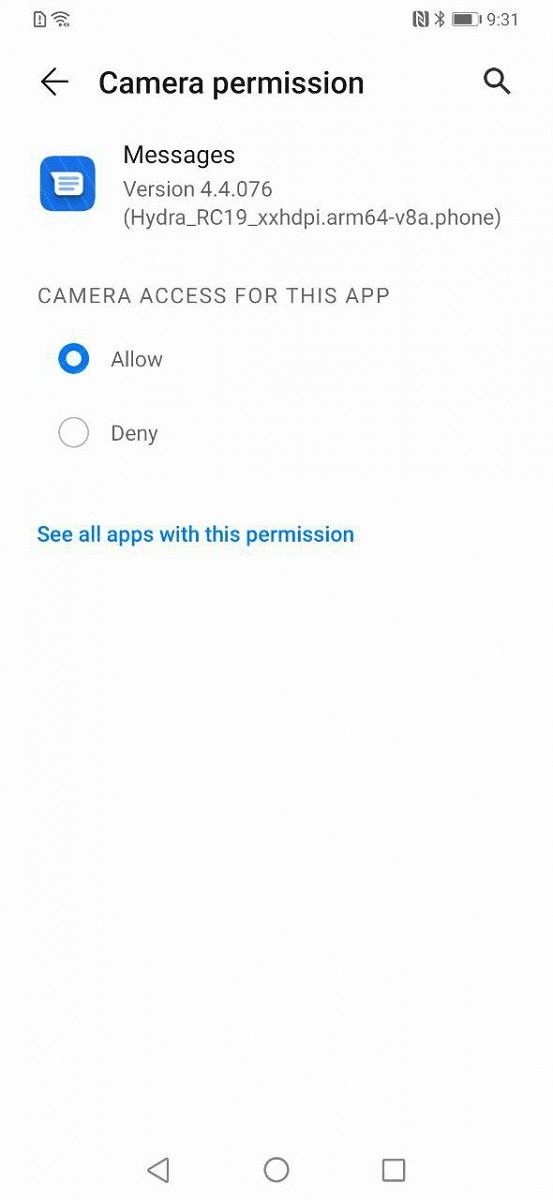The image depicts a screen requesting permission to access the camera for a specific application. The prompt offers a choice to either allow camera access for this instance or deny it. Unlike general permission requests that apply to all apps, this one is specific to the originating app, which appears to be a messaging application. The text reads: "Messages version 4.4.076," with additional details in brackets: "Hydra (H-Y-D-R-A)_R-C-19_XXHDPPL.arm (A-R-M-64) version 4.4.076." This detailed string is repeated within the prompt.